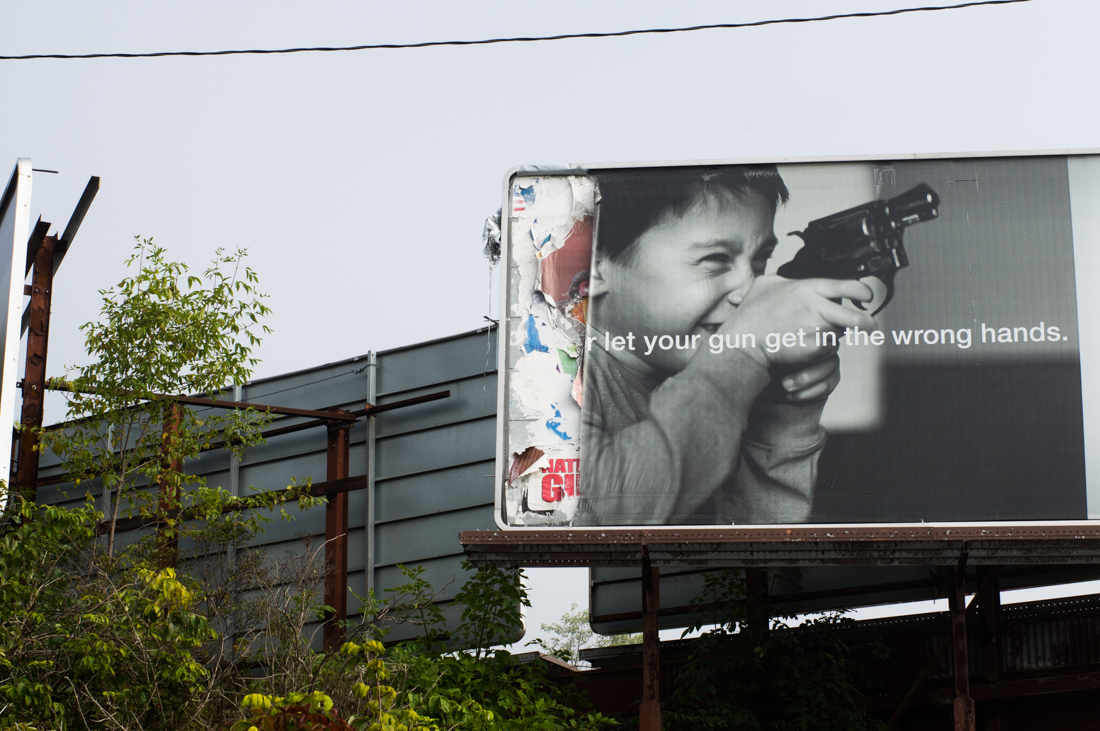The photograph depicts a prominently positioned billboard with a slightly rounded rectangular shape. The main feature of the billboard is an image rendered in shades of black and gray, depicting a young child holding a black revolver-style firearm. The accompanying text on the billboard reads: "Let your gun get in the wrong hands." The billboard appears damaged, with a portion missing, revealing old, ripped-up advertisements behind it. In the background, the scene includes the backs of other metal billboards or signs, and there's visible greenery, particularly on the left side, where trees and leaves protrude into the frame. A gray, overcast sky covers the background, intersected by a power line that stretches across the top of the image.